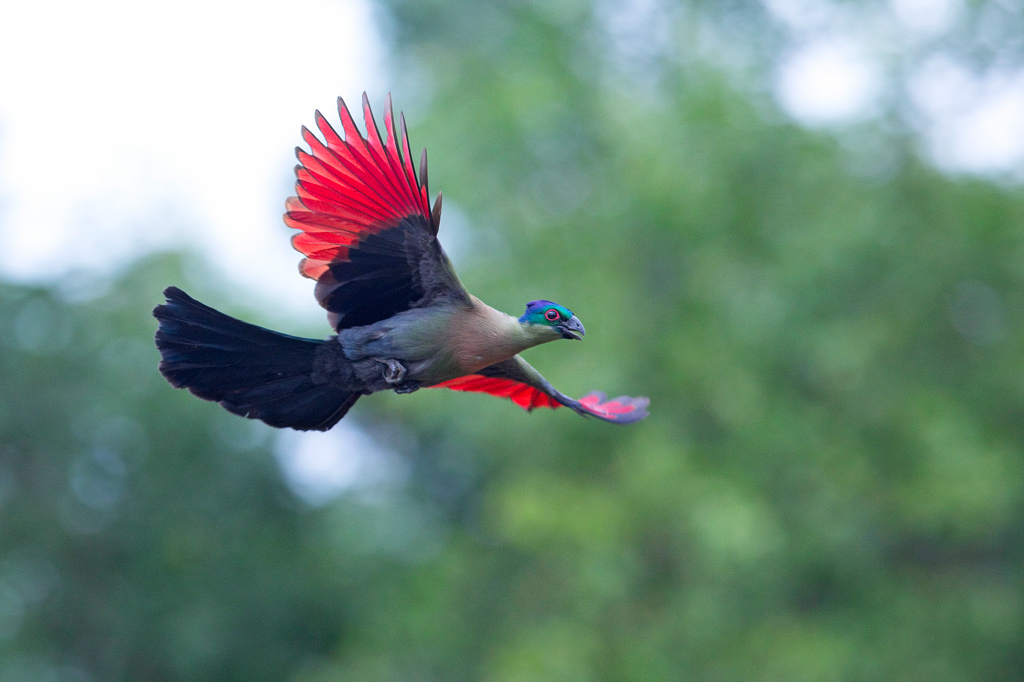In this stunning rectangular photograph, the central focus is a vibrant, small bird mid-flight against a blurred background suggesting lush green foliage. The bird's detailed plumage showcases a captivating mix of colors: its stomach is a gradient of gray and blue, while its neck and back are pristine white. The underside of its head is a striking blue, ornamented with dark blue, turquoise, and black spots. Its impressive wings are fully outstretched, marked by red tips contrasting with black feathers. The tail feathers echo the blue and black theme.

Its distinctively short black beak and large, expressive red-and-black eyes are particularly eye-catching. The bird's legs are neatly tucked into its body, revealing three black claws on each. This photograph captures the bird's vibrant hues and complex textures, making it appear almost otherworldly, like a modern-day descendant of dinosaurs. The close-up nature of this photograph allows viewers to appreciate the bird's natural beauty and the soft-focus background enhances its remarkable presence in what appears to be its natural habitat, possibly in Sub-Saharan Africa.